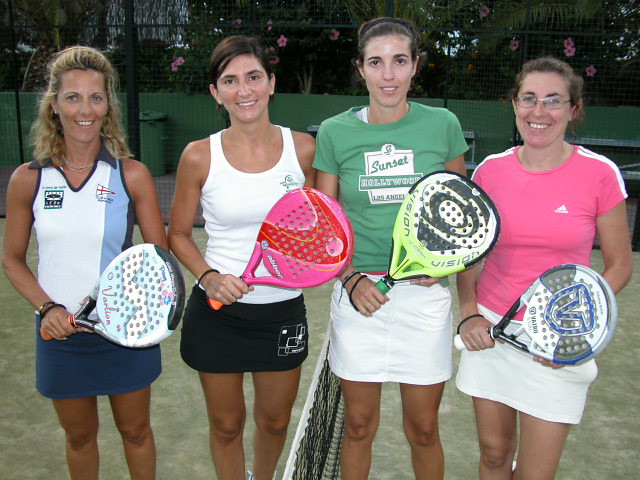The photo captures four middle-aged women posing with pickleball paddles on an outdoor court. They are standing in front of a net, which suggests they had been playing a 2v2 game. The women are all facing the camera and smiling warmly. 

One woman is dressed in a white and light blue collared shirt paired with a blue skirt, another is wearing a white tank top with a black skirt. The remaining two women are dressed in white skirts; one sports a green t-shirt, while the other wears a pink Adidas t-shirt. 

The court appears to have a worn artificial grass surface. In the background, there is a green walkway with benches, some greenery, and pink flowers, indicating a well-maintained area. This lively summer scene effectively captures the essence of recreational pickleball and camaraderie.